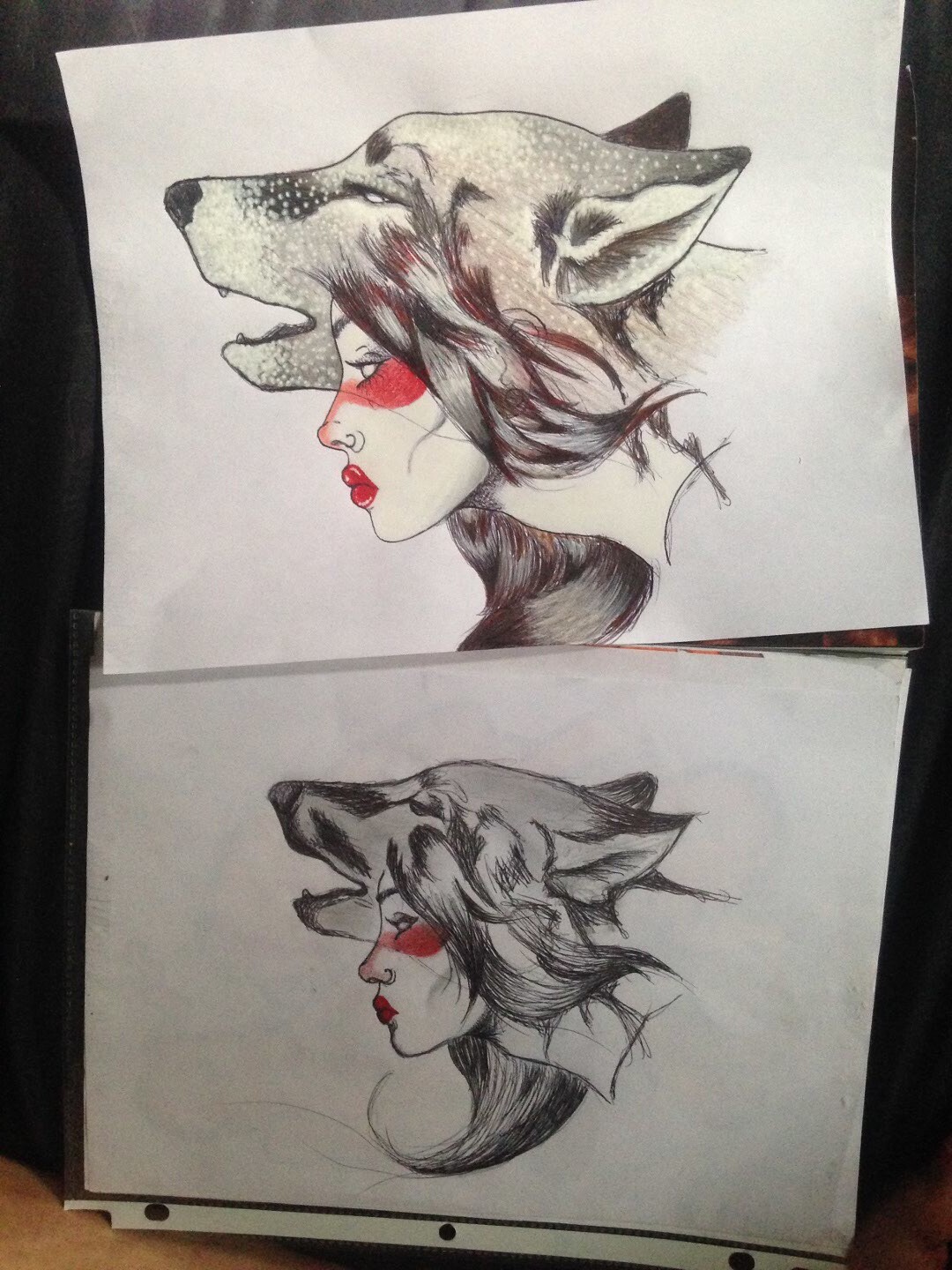In this image, there are two drawings displayed one above the other. The bottom drawing, enclosed in a three-hole punched plastic sleeve, appears to be a reference image or initial sketch. It features a woman's face adorned with a wolf's head. The woman has black hair cascading down, red lips, and red accents beneath her eyes and on her nose. The wolf's head, depicted in dark shades, has closed eyes and ears that are pulled back, painted in a mix of gray and dark black hues. Notably, the woman's neck extends backward rather than downward from her face.

The top drawing is a more refined and detailed version of the same image. The wolf's fur is rendered with greater intricacy, including speckled white dots, giving it a more lifelike texture. The woman's face and eyes are also depicted with much finer details, enhancing the overall realism and depth of the artwork.